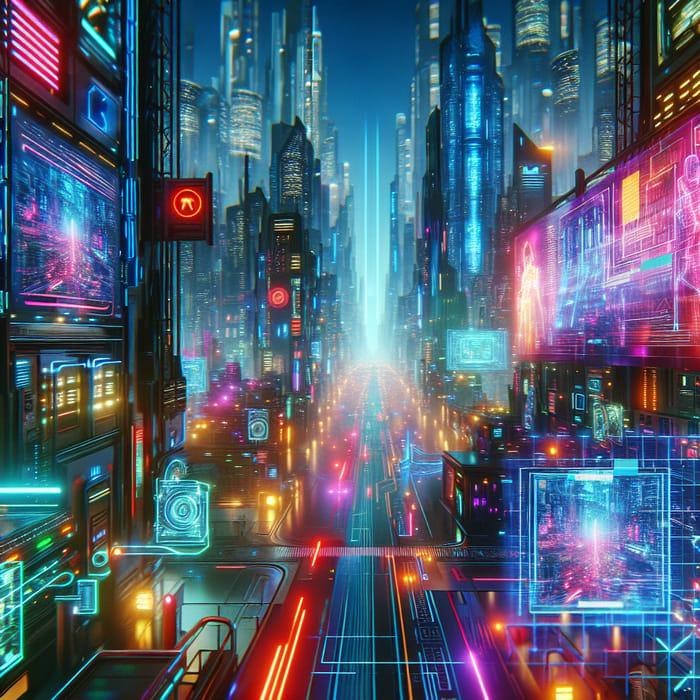This digital illustration captures a futuristic, cyberpunk cityscape reminiscent of Blade Runner. The scene is depicted in a wide vertical format, showing a nighttime street flanked by tall skyscrapers adorned with vibrant neon signs and holographic advertisements. Motion lines on the street suggest fast-moving vehicles, with beams of light stretching across the scene. The color palette is dominated by blues, purples, and red-oranges, creating an electrified, almost surreal atmosphere. The sky, though barely visible through the dense array of high-rise buildings, retains a tinge of blue, contrasting the heavily illuminated street. Notably, the image is devoid of people, emphasizing the architecture and technological elements. In the bottom right corner, a detailed glimpse inside a building room enhances the sense of looking into a meticulously crafted, computer-generated metropolis.